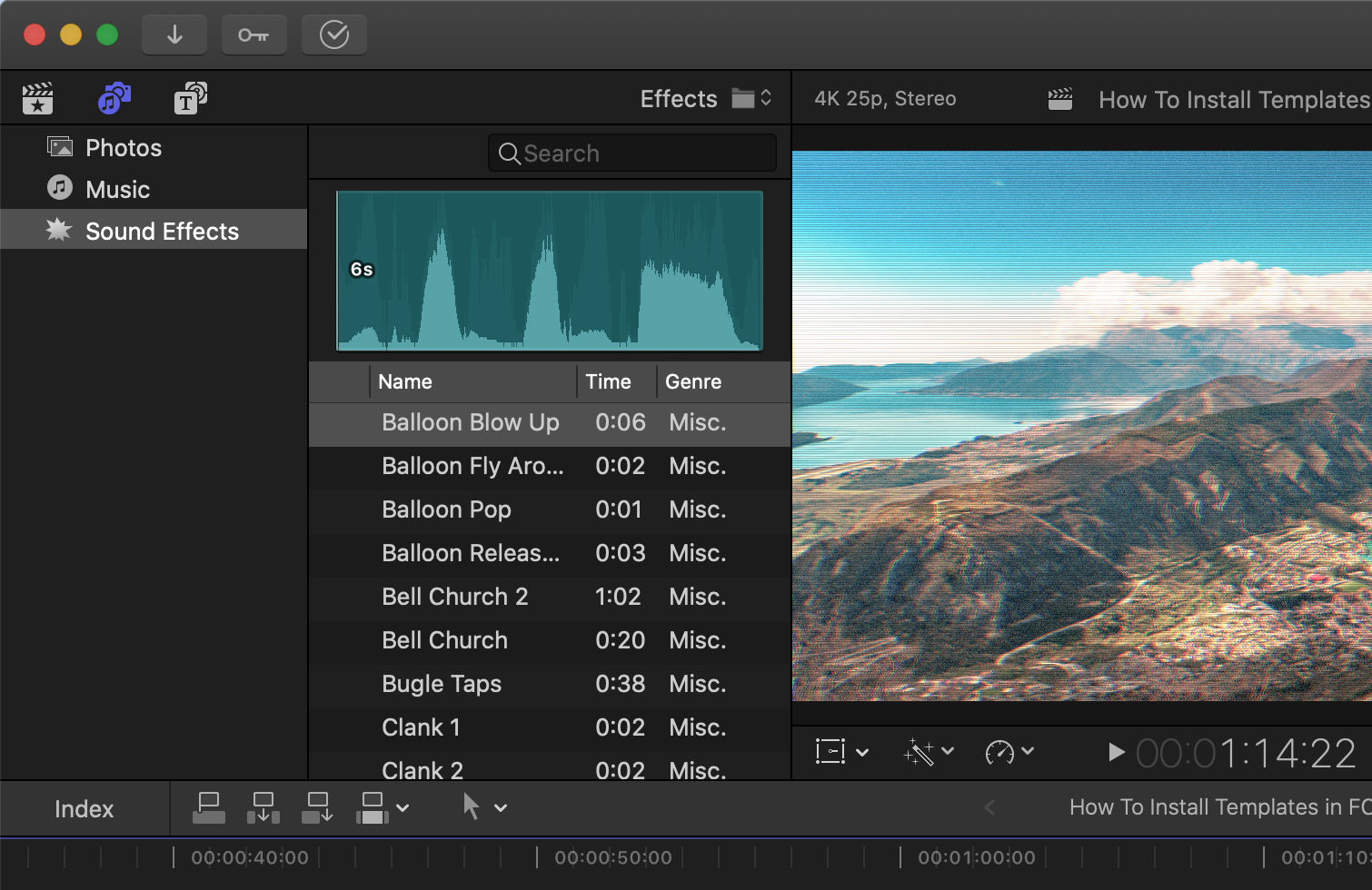The interface of the image in question is quite detailed and presents various elements organized in distinct sections. At the top, there's a gray border that encapsulates three colored circles: one red, one yellow, and one green. To the right, it also boasts buttons including one with a downward arrow and another with a circle and a check mark.

On the left side, there's a vertical sidebar featuring categories such as Photos, Music, and Sound Effects. Following this, there is a search box containing terms like 'effects', '4k', '25p stereo', and 'how to install templates'. Adjacent to the sidebar is a graph, represented in blue and resembling sound waves, adding a dynamic visual element, though its exact purpose is unclear.

The main content area displays a picturesque image capturing a serene scene with water, looming mountains, a blue sky adorned with clouds. Overlaying this image is tabular information, divided into columns labeled 'Name', 'Time', and 'Genre'. The listed items include audio clips with names and detailed durations such as:

- Balloon Blow Up: 6 seconds, Miscellaneous
- Balloon Fly A-R-O...: 2 seconds, Miscellaneous
- Balloon Pop: 1 second, Miscellaneous
- Balloon Release: 3 seconds, Miscellaneous
- Bell Church 2: 1 minute, 2 seconds
- Bell Church: 20 seconds

The genre for most sound effects is marked as Miscellaneous, providing a categorized, time-specific overview of the available audio clips in the interface.